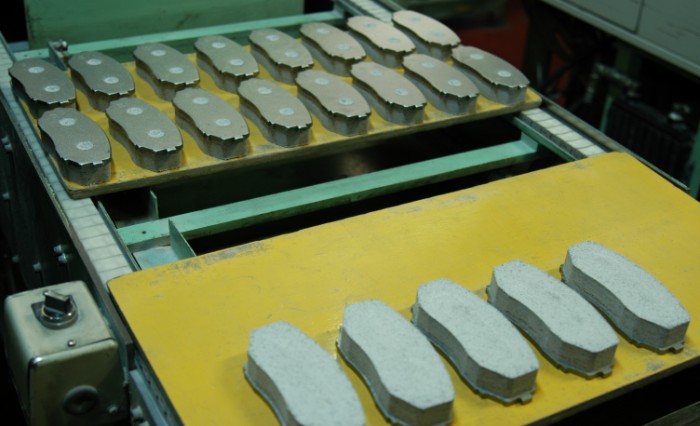The image depicts a close-up view of a large, industrial metallic machine, specifically focusing on its conveyor belt and various attached components. The conveyor belt is primarily constructed from dark gray steel and is accompanied by a control panel with a black knob, likely used to adjust the conveyor's speed. A noteworthy feature is the green horizontal bar that connects the machine’s steel frame, providing structural support.

Central to the image are two prominent yellow slabs or plates positioned at different points on the conveyor belt. The first yellow slab on the right has five small, coffin-shaped metal plates arranged side by side. Conversely, the slab on the left holds 16 similar metal plates, arranged in two rows of eight, but these are displayed flipped over, revealing smooth undersides with two circular indentations each. The overall machinery also appears interspersed with metal bolts and gears, suggesting an intricate, mechanical setup, possibly for manufacturing or molding processes related to the metal plates.